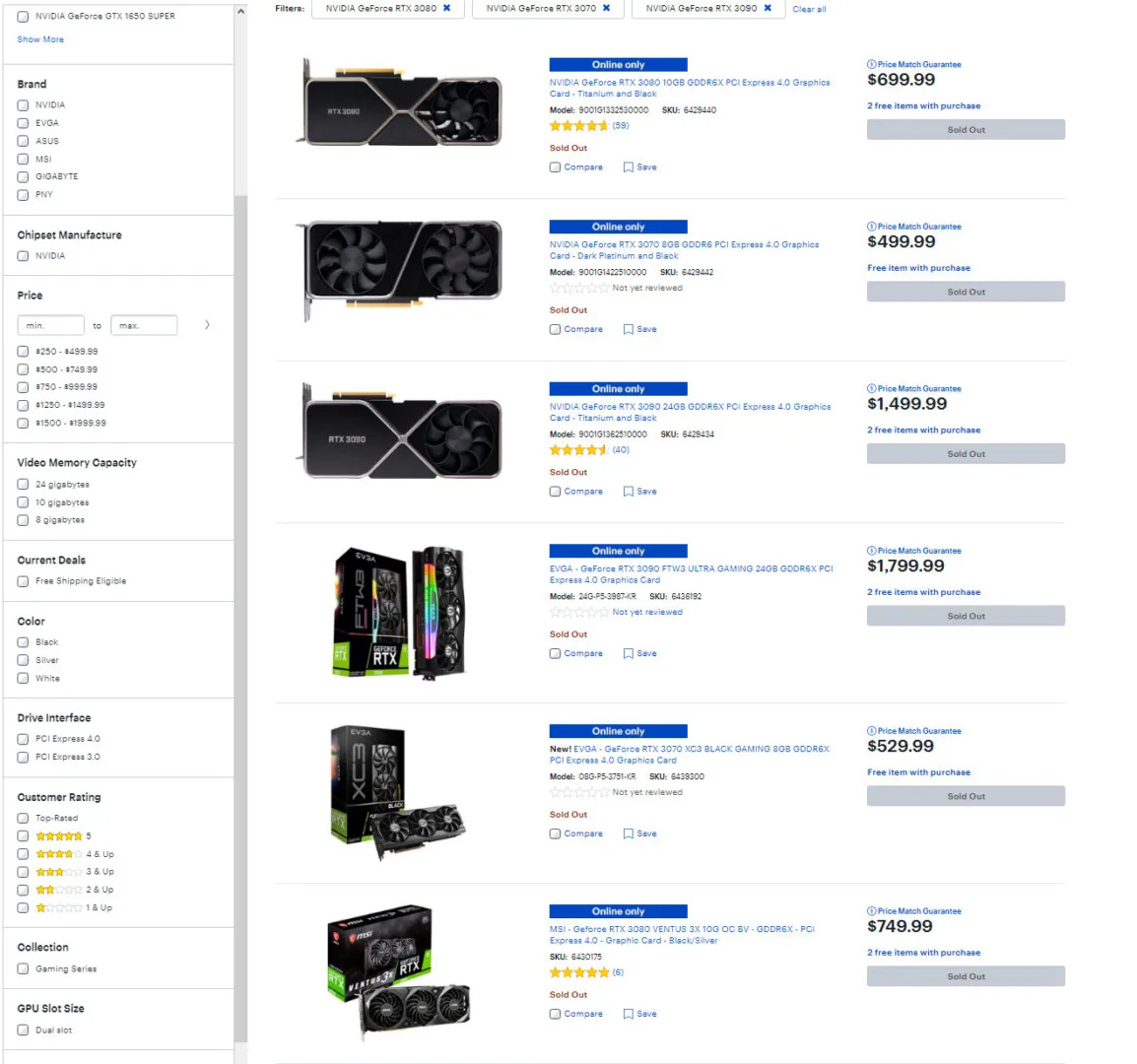The image showcases an online shopping catalog specifically for computer graphic cards. The website features a clean white background with black text for easy readability. Each product has a gray button labeled for purchasing or obtaining more information, alongside blue text that details the item description and provides a clickable link to the product page. 

On this page, six different graphic cards are prominently displayed:
1. The first graphic card is priced at $699.99.
2. The second graphic card is available for $499.39.
3. The third graphic card, one of the higher-end options, is listed at $1,499.99.
4. The fourth graphic card is the most expensive, with a price tag of $1,799.99.
5. The final graphic card on the main section of the page is offered for $529.39.
6. At the very edge of the page, another graphic card is visible, priced at $749.99.

The structured layout and systematic presentation of prices and links make it easy for customers to navigate and select the desired graphic card for their computer needs.